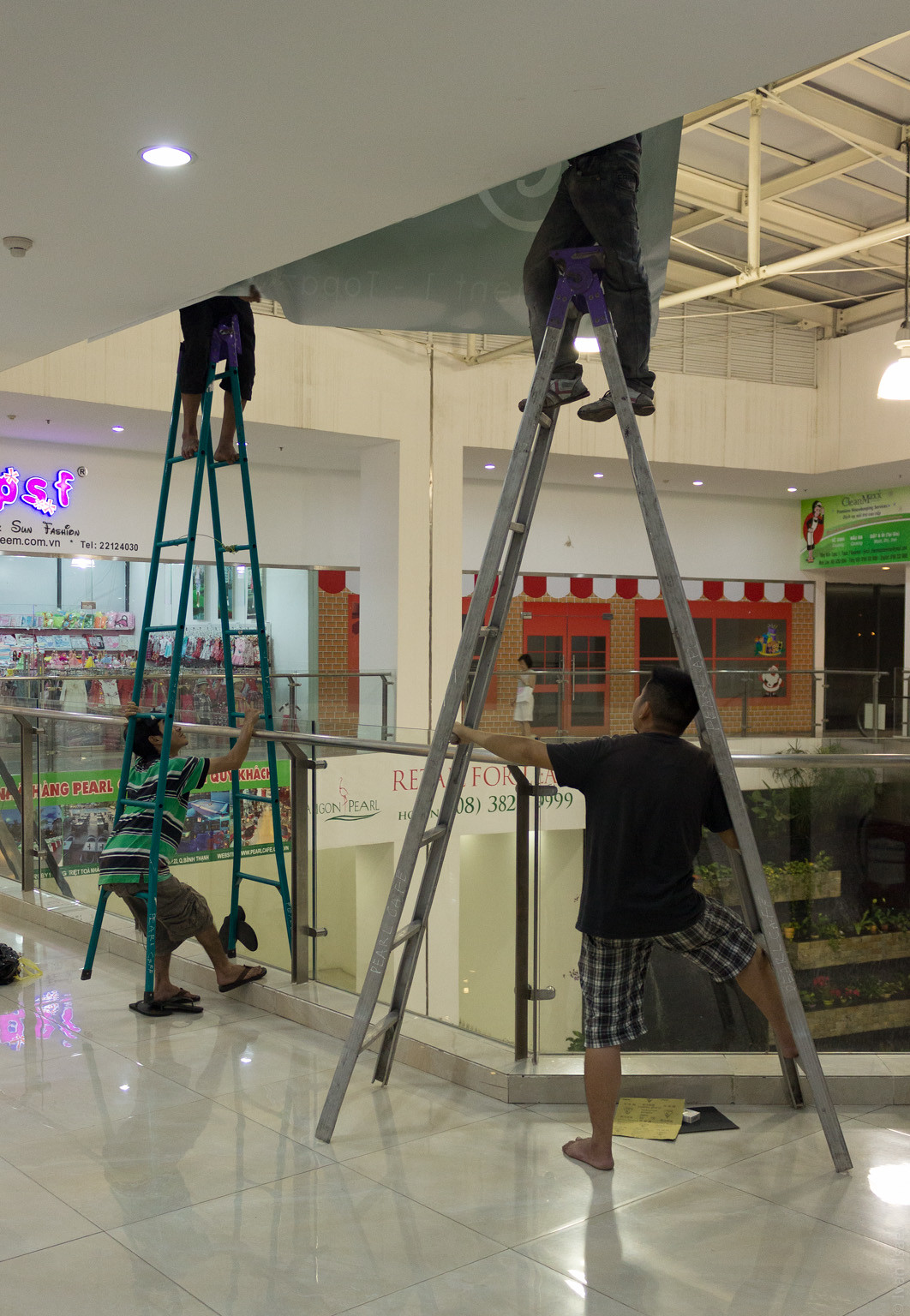This photo, taken inside a two-story shopping mall, captures a busy scene on the second floor. In the background, you can see stores, one distinguished by double doors topped with a white and red banner. The foreground reveals a white tiled area bordered by glass walls and railings, offering a view down to the lower level. Two ladders are set up in front of the railing: a green one on the left and a silver one on the right. Each ladder is held steady by a man; the one on the left wears a black and green striped shirt, shorts, and flip-flops, while the one on the right is in a black shirt, checkered shorts, and no shoes. At the top of each ladder, only the legs of the men doing the work are visible; they balance precariously, with one on the purple bench of the ladder, dressed in long black pants and shoes. The scene suggests they are hanging a banner, emphasizing the height above the first floor and the care taken to ensure safety.